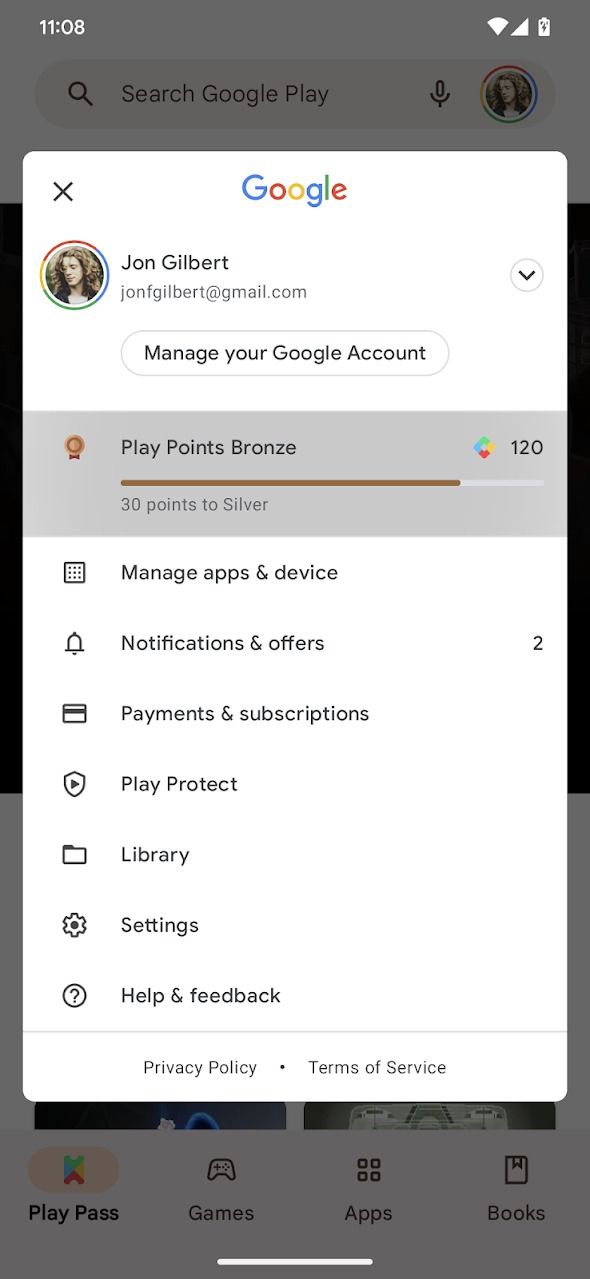The image features a gray background with the time displayed as 11:08. At the top, there's a battery icon showing a charging symbol. Below this, a search bar labeled "Search Google Play" appears, accompanied by a magnifying glass icon on the left and a microphone icon on the right. On the far right, there is a profile picture with the label "John Gilbert" and an email address "JohnFGilbert@gmail.com".

An oval button marked "Manage your Google Account" is present. Underneath, a gray rectangle shows "Play Points" with the status indicating "Bronze: 30 points to Silver: 120". Below this section, several options are listed including "Manage apps and device," "Notifications and offers," "Payments and subscriptions," "Play Protect," "Library," "Settings," "Help," and links to the "Privacy Policy", and "Terms of Service."

The lower section of the image features tabs labeled "Play Pass," "Games," "Apps," "Movies & TV," and "Books," with the "Play Pass" tab highlighted in pink. At the bottom middle, there is a white horizontal bar.